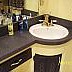The image depicts a close-up view of a bathroom countertop area. The square frame measures approximately 2.5 inches by 2.5 inches, capturing a small and detailed scene. Dominating the right side of the image is a circular white sink, which appears to be fairly shallow. The sink is complemented by a gold faucet in the center with two side handles, likely for regulating temperature and water flow.

The countertop itself is a very dark brown, creating a stark contrast against the white sink and the gold fixtures. Beneath the countertop, there is a beige cabinetry setup. Notably, there is a dark brown square area beneath the sink, possibly a cutout or part of the cabinet design, and to the left of it, a rectangular drawer with a silver handle.

In the background, the upper right corner reveals a yellow-colored wall, adding a splash of color to the scene. In the upper left corner of the sink area, various bottles are visible; some are clear while others have a blue tint. These bottles could contain lotions or other bathroom essentials. The overall composition of the image suggests a stylish yet functional bathroom sink setup.